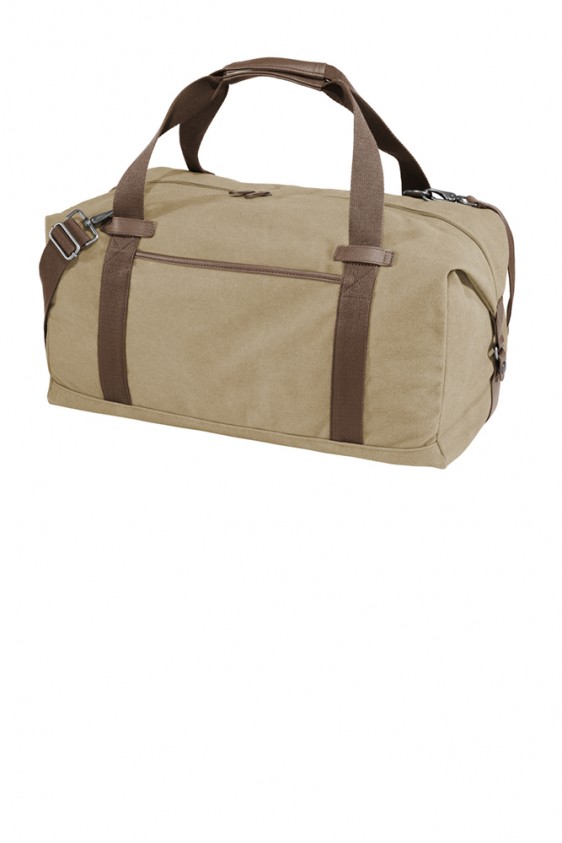This is a detailed description of a beige canvas duffel bag, viewed from the side and appearing full. The bag features two short, dark brown handles with a Velcro or leather grip to connect them for easier holding, along with a long, detachable shoulder strap, also in dark brown. The bag is equipped with buckles on either end for added security and versatility. Metallic silver hooks fasten the straps. The duffel has a main zipper that spans the entire top length, opening the bag, and a small pouch on the front for additional storage. No distinctive lettering is visible on the bag, except for a faint mark near the top, and overall, it maintains a minimalistic design without other prominent colors.